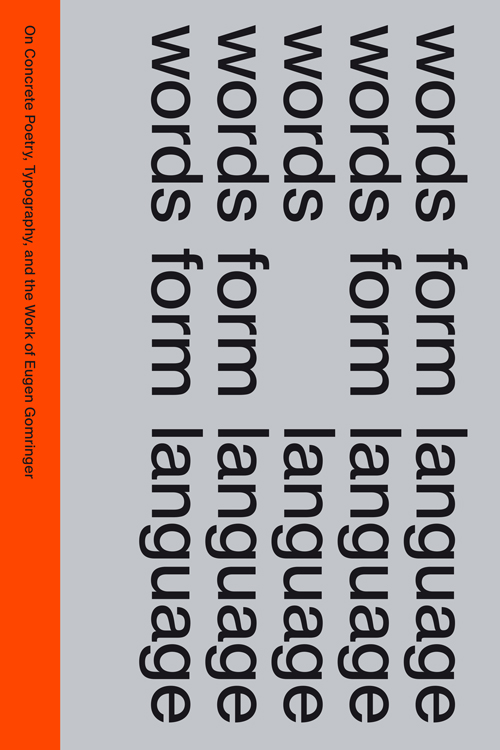The rectangular image, approximately six inches tall and four inches wide, features a light blue-gray background with five rows of black lettering arranged vertically. The text on each row reads “words form language” except for the third row, which simply says “words    language,” missing the word “form” in the center. A vertical orange bar spans from top to bottom on what would be the bottom of the image when viewed correctly, but it appears on the left side due to the image being rotated. The black text within this bar reads "On Concrete Poetry, Typography, and the Work of Eugene Gomringer," referring to the famed concrete poet, extending about half an inch from the former bottom left corner.